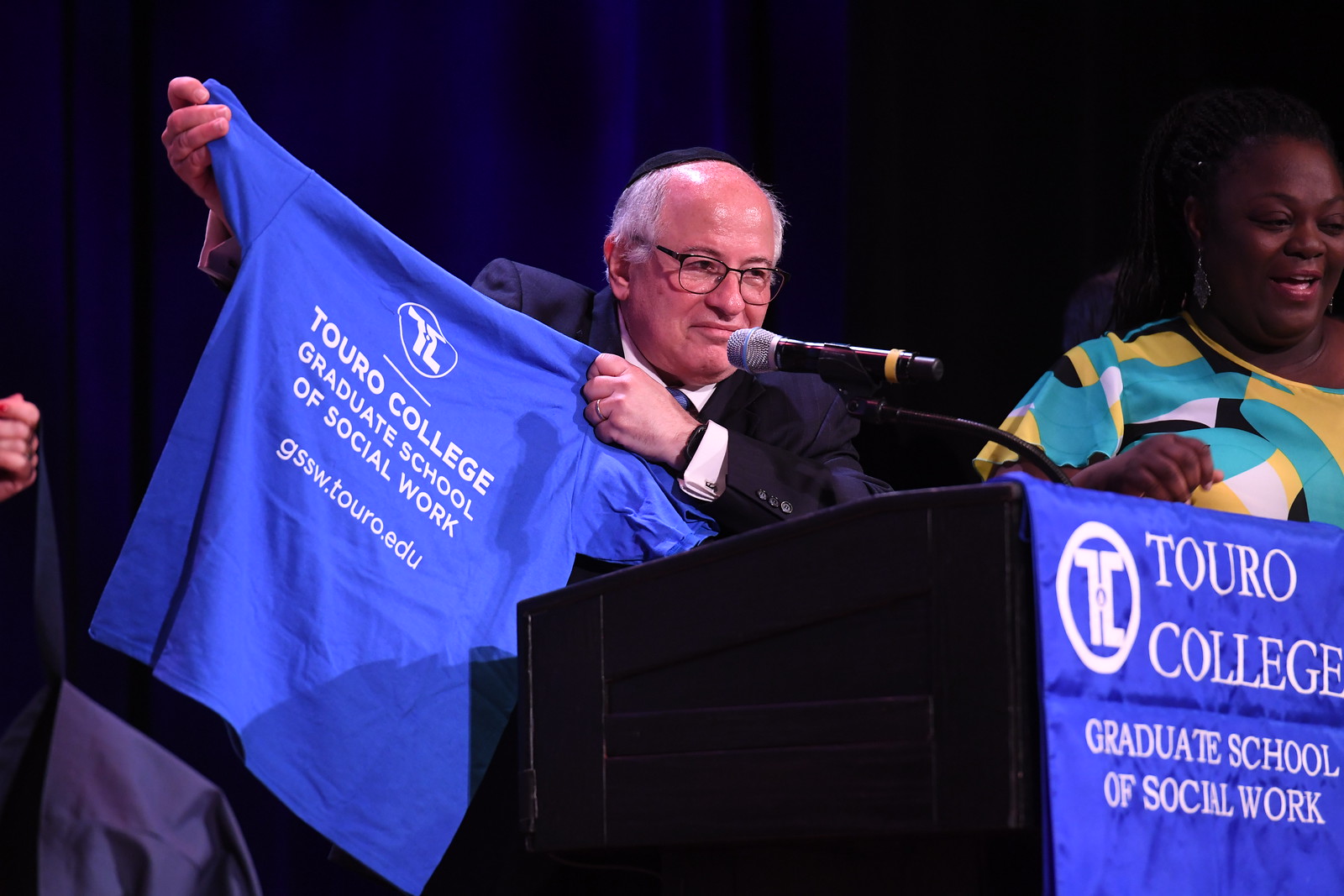In this detailed indoor image set within a college during what appears to be a presentation or award ceremony, an elderly man, centered in the frame, stands behind a dark-colored podium adorned with a blue banner. The banner prominently displays the text "Toro College Graduate School of Social Work" in a serif font, accompanied by the college logo. The man, distinguished by his bald top, black-framed glasses, and white hair around his ears, speaks into a black microphone that features a gold band. He is dressed in a suit and holds a blue t-shirt in his right hand, outstretched to display its white lettering that reads "Toro College Graduate School of Social Work" followed by "gssw.touro.edu" in a sans serif font. Behind him is a vertically pleated blue curtain. To the right side of the image, a black woman is visible, smiling and looking towards something off-camera. The color palette of the image includes black, blue, white, light blue, yellow, brown, gray, and tan.